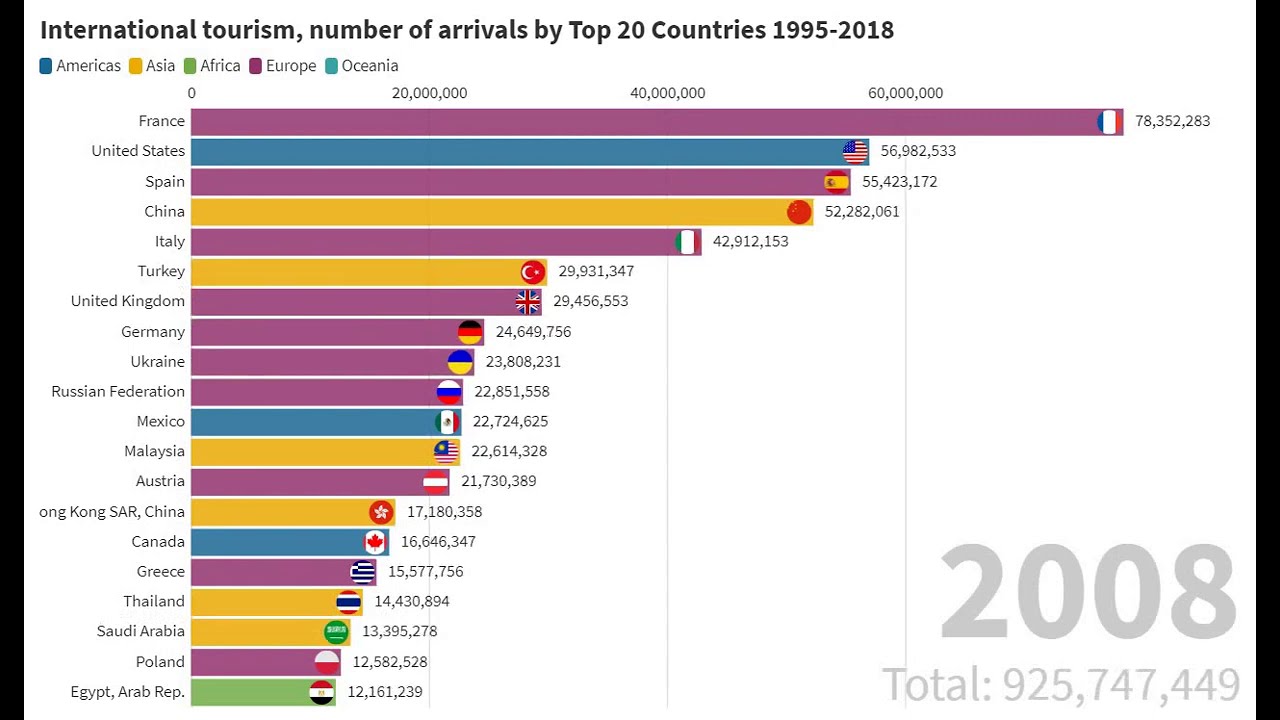The image showcases a detailed line chart titled "International Tourism: Number of Arrivals by Top 20 Countries (1995 to 2018)" in black letters at the top. The chart, set against a white background, features a color-coded key indicating that blue represents the Americas, yellow represents Asia, green represents Africa, pink represents Europe, and teal represents Oceania. Each country is listed with corresponding lines that trace the number of tourist arrivals over the given period, complete with the country's flag at the end of each line. Prominently, the lower right-hand corner shows the year "2008" in large light gray letters, alongside the total number of arrivals: 925,747,449. Notable countries listed on the chart include France, the United States, Spain, China, and others, all highlighted with colored lines corresponding to their respective regions. The clean and structured layout, with an emphasis on clear and distinguishable colors, suggests that this chart could be used in a professional setting, such as a PowerPoint presentation.